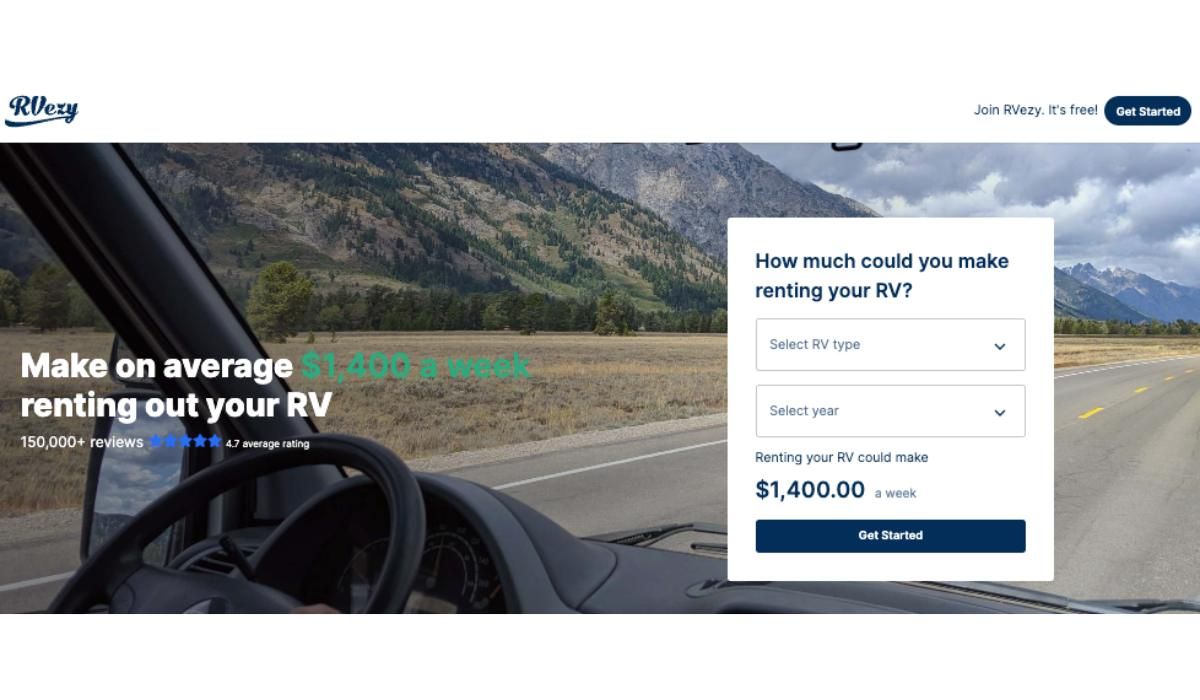This is a cropped screenshot from the RVZ website. In the top-left corner, the RVZ logo is prominently displayed. On the top-right, there's a call to action encouraging viewers to "Join RVZ. It's free," followed by a striking blue button labeled "Get Started." Below this header is a large, captivating photo that serves as the background, depicting a scenic view from inside an RV as it travels down a road with a mountain range in the distance.

On the far left within the image, text in white reads "Make on average $1,400 a week renting out your RV," with the figure "$1,400 a week" highlighted in green for emphasis. Beneath this, a testimonial statistic states "150,000+ reviews, 5 stars, 4.7 average rating," with the stars icon colored blue. 

To the right of this photo background is a prominent white box that poses the question "How much could you make renting out your RV?" in dark blue font. Below this query are two drop-down selection boxes, one for "Select RV type" and the other for "Select year." At the bottom-left corner of this section, it reiterates that "renting your RV could make $1,400 a week," and another "Get Started" button is placed at the very bottom to encourage action.